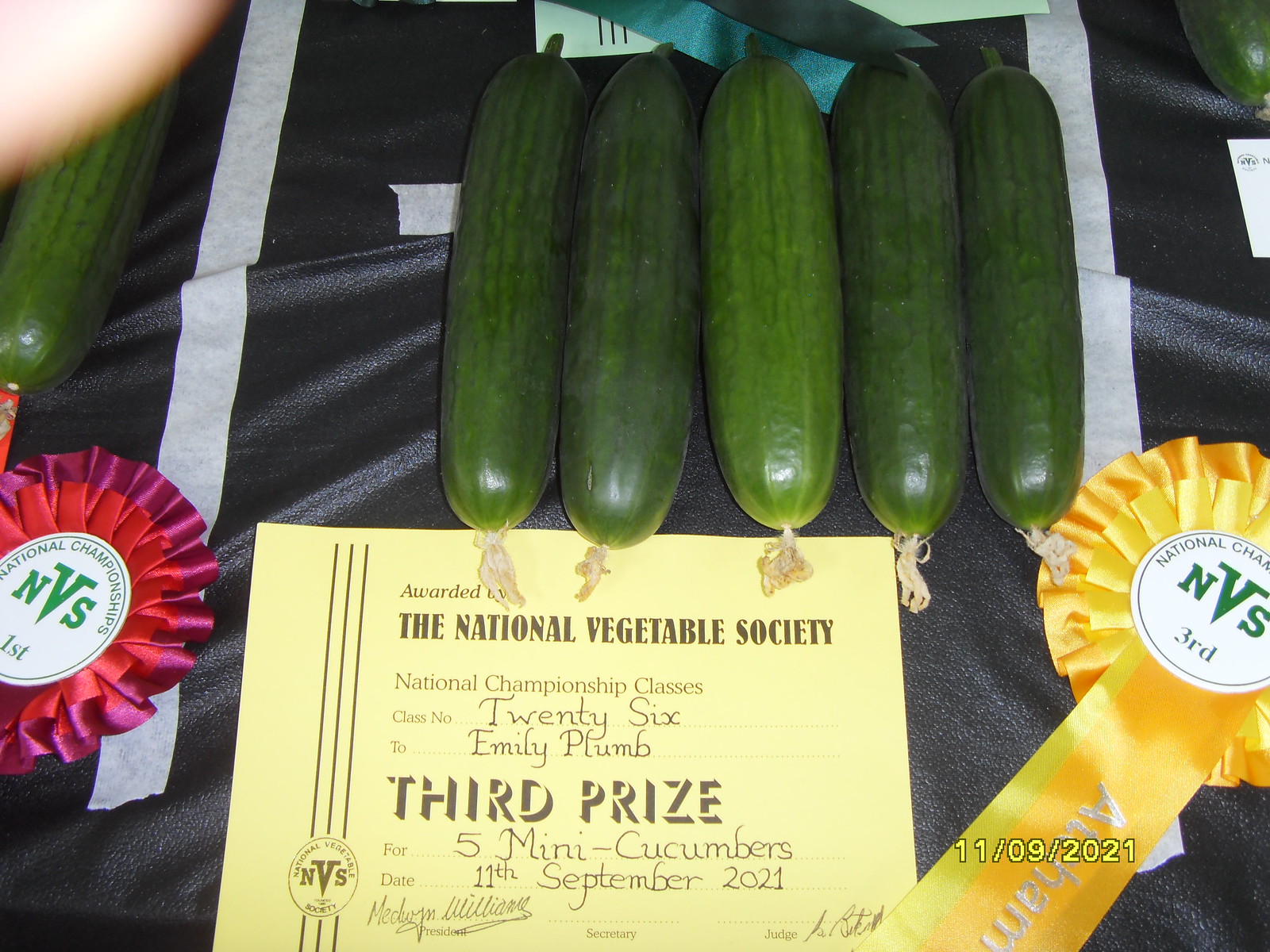The image features five shiny, green mini cucumbers neatly arranged on a black, shiny tablecloth with white lines. A cream-colored card in front of the cucumbers states that they were awarded third prize by the National Vegetable Society at the National Championship Classes, class number 26, to Emily Plum. The date on the card reads September 11, 2021. On the left side of the image, partially visible, is a red ribbon awarded to another set of cucumbers, denoting a first prize. Towards the bottom right of the cucumbers, a yellow ribbon marks the third prize won by Emily Plum. The black tablecloth has strips of tape that divide the entries.